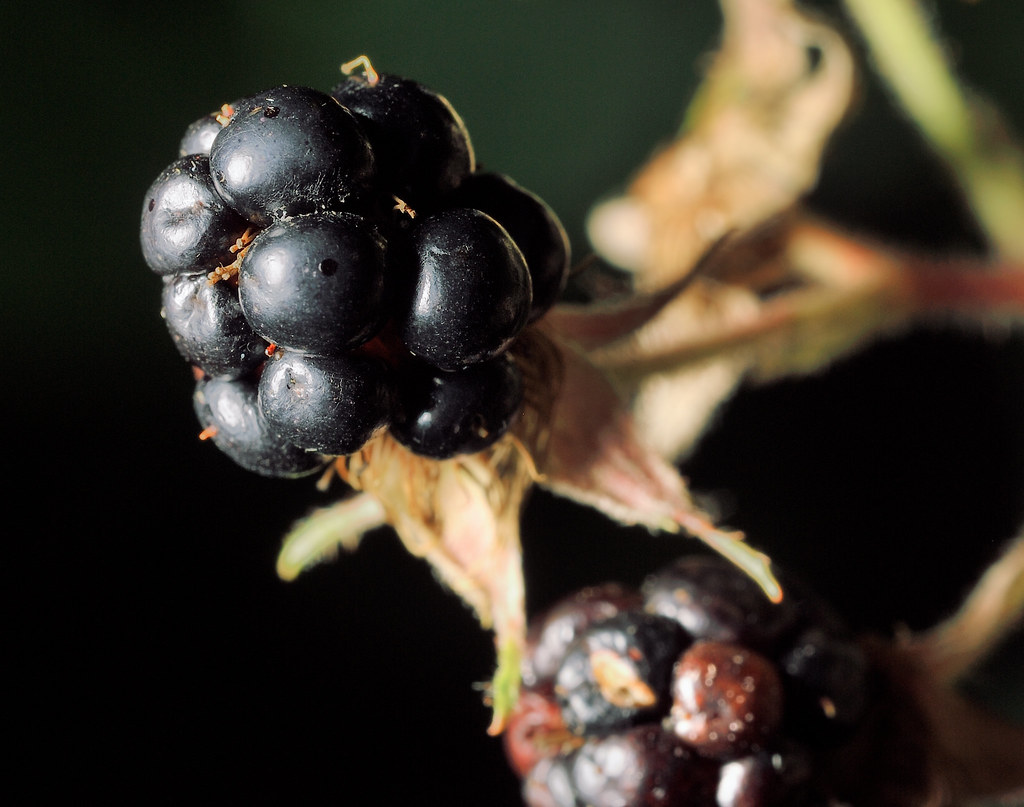This high-resolution, professional photograph captures an up-close view of a cluster of dark navy to black berries, possibly blackberries or a similar type of fruit. Each individual berry is ripe and boasts a rich, purplish-black hue. The main cluster is the focal point of the image, prominently displayed against a dark black background. One of the berries in the foreground appears slightly damaged, revealing a tan interior that resembles the texture of a grape or blackberry. The cluster is supported by yellowish-green stems, and additional berries can be seen below, though they are out of focus. In the blurred background, the leafy part of the plant adds a green contrast, emphasizing the vivid details of the berries.